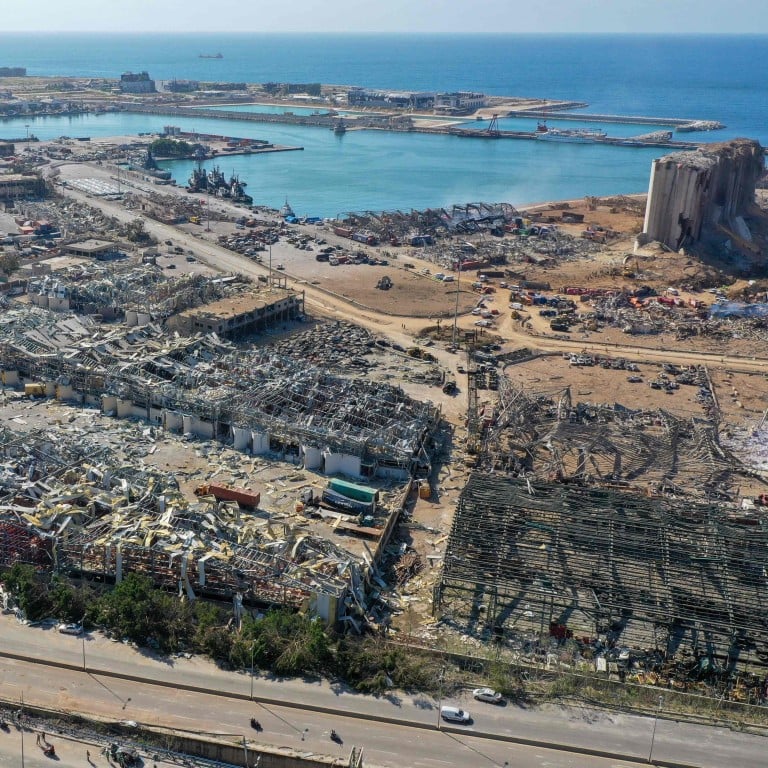This aerial photograph reveals the devastated aftermath of a large-scale explosion in a coastal city, likely Beirut. The scene is dominated by widespread destruction: numerous buildings are completely ruined, with some high-rise structures visibly toppled or severely damaged. The foreground shows a road lined with burnt-out cars and debris, while the middle ground is cluttered with a mix of metal lattices, shredded fabric, and other unrecognizable fragments of infrastructure. A modern harbour, central to the image, exhibits melted roofs and flattened structures, testifying to the intensity of the blast—presumably the infamous 2020 Beirut explosion caused by improperly stored ammonia nitrate. The turquoise blue sea forms a stark backdrop to the chaos, extending to the horizon with a long boat floating near it. The once-thriving coastline is now marked by its displaced, sunlit ruins, with no visible traces of human life left in the photograph.